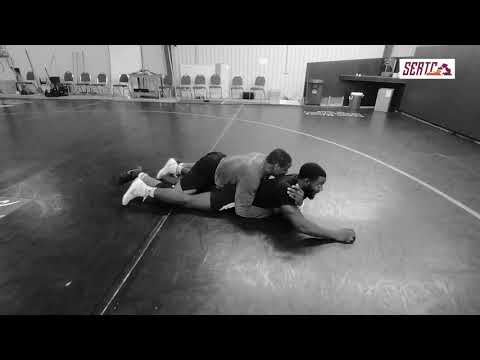This black and white image captures an intense wrestling match between two men on a wrestling mat. The man on the bottom, dressed in a black shirt, black shorts, and white shoes, is laying on his stomach with one arm extended far out in front of him. On top of him, a second man, wearing a gray shirt, black pants, and black shoes, has his arms wrapped firmly around the other man's torso. Both wrestlers have dark black hair and are facing to the right. The mat they are on features a prominent half-circle design extending from the bottom right to the top left. In the background, there's a white, rippled wall lined with chairs. In the top right corner of the image, a small label reads "S-E-R-T-C" with an emblem of two people wrestling next to it. The setting appears to be a gymnasium, possibly a multi-purpose sports venue.